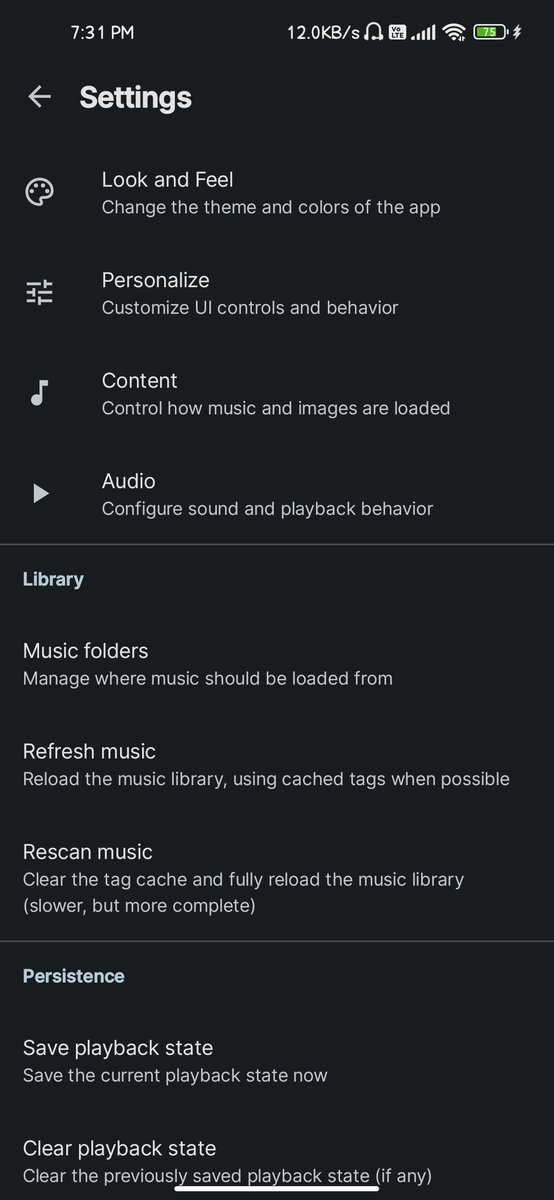The screenshot displays a cell phone screen against a solid black background. In the upper left corner, the time is shown as 7:31 PM. In the upper right corner, the status icons indicate full signal bars, Wi-Fi connectivity, and a battery at 75% charge. Below, in bold white text, is the heading "Settings" with a left-pointing arrow beside it. 

Beneath the main heading, several menu items are listed with brief descriptions:
- "Look and Feel": Allows changes to the theme and colors of the app.
- "Personalize": Lets users customize the UI controls and behavior.
- "Content": Provides options for controlling how music and images are loaded.
- "Audio": Contains settings for configuring sound and playback behavior.

A thin, light gray horizontal line separates these settings from additional options further down:
- "Library": Includes settings for managing where music should be loaded from.
- "Music Folders": Offers control over the directories used for music storage.
- "Refresh Music": Describes reloading the music library using cached tags when possible.
- "Rescan Music": Details the process of clearing the tag cache and fully reloading the music library, noting that this option is slower but more comprehensive.
- "Persistence": Provides options to save and clear the playback state.

This descriptive caption covers all the details visible in the screenshot.